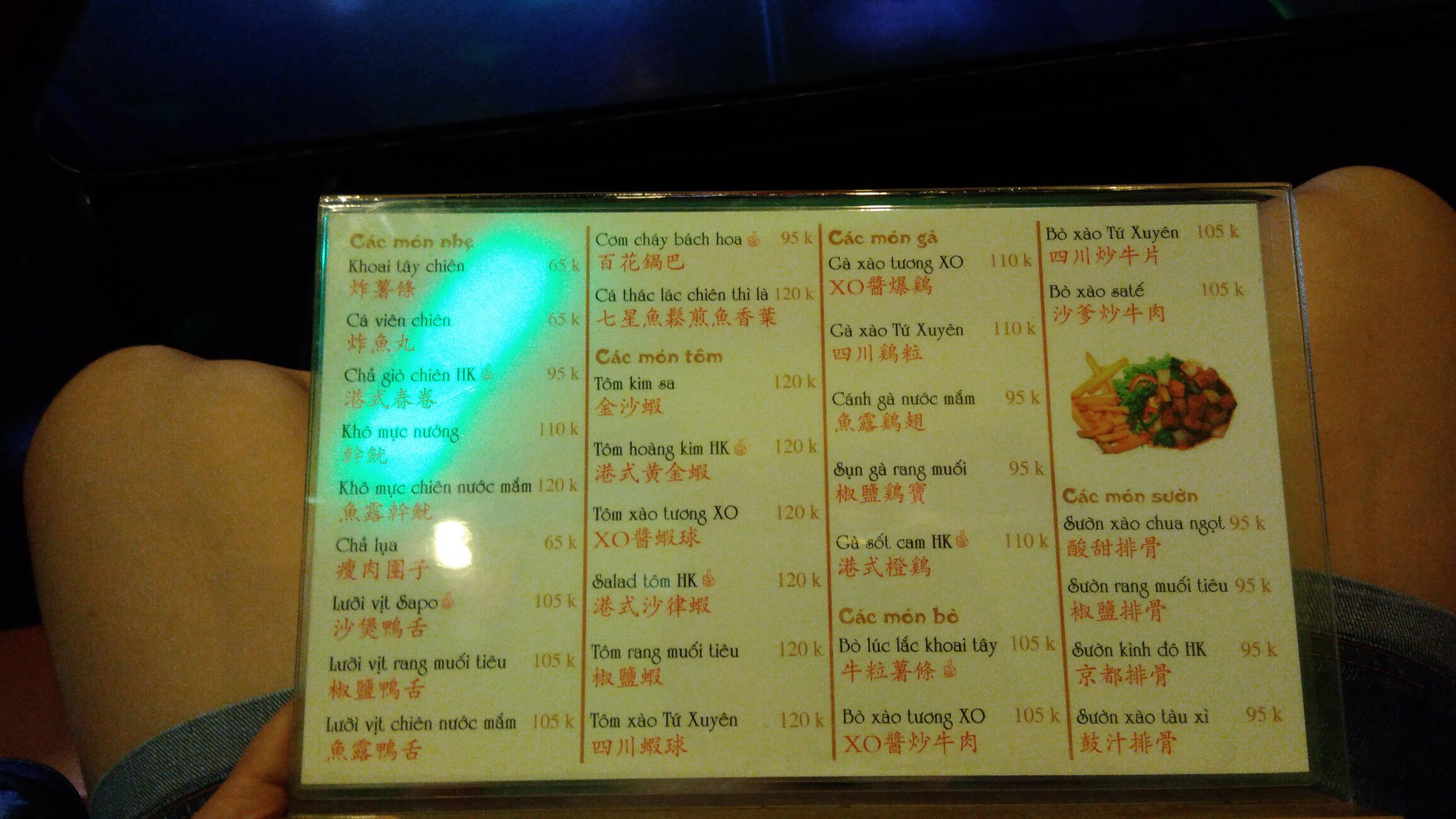In this landscape-oriented photograph captured from a first-person perspective, the viewer is immersed in a scene where an individual is holding a food menu. The person's legs are visible, clad in blue denim shorts, contributing to the casual ambiance of the setting. The menu occupies the central focus of the image, illuminated by a gleam of light in the upper left corner, which softly highlights its details. The menu is bilingual, featuring both English and what appears to be Mandarin or Chinese characters. 

Prominent categories on the menu include "Kok Mon Og," "Kok Mon Cho," "Kok Mon Ga," and "Kok Mon Suon," though the foreign script provides depth to the textual arrangement. Prices are displayed on the right side, with the currency marked as 'K', displaying denominations such as 120K, 65K, 105K, and 95K. These details, though small and subtly lit, suggest a varied and intriguing selection of dishes, inviting the viewer to explore the culinary offerings further.